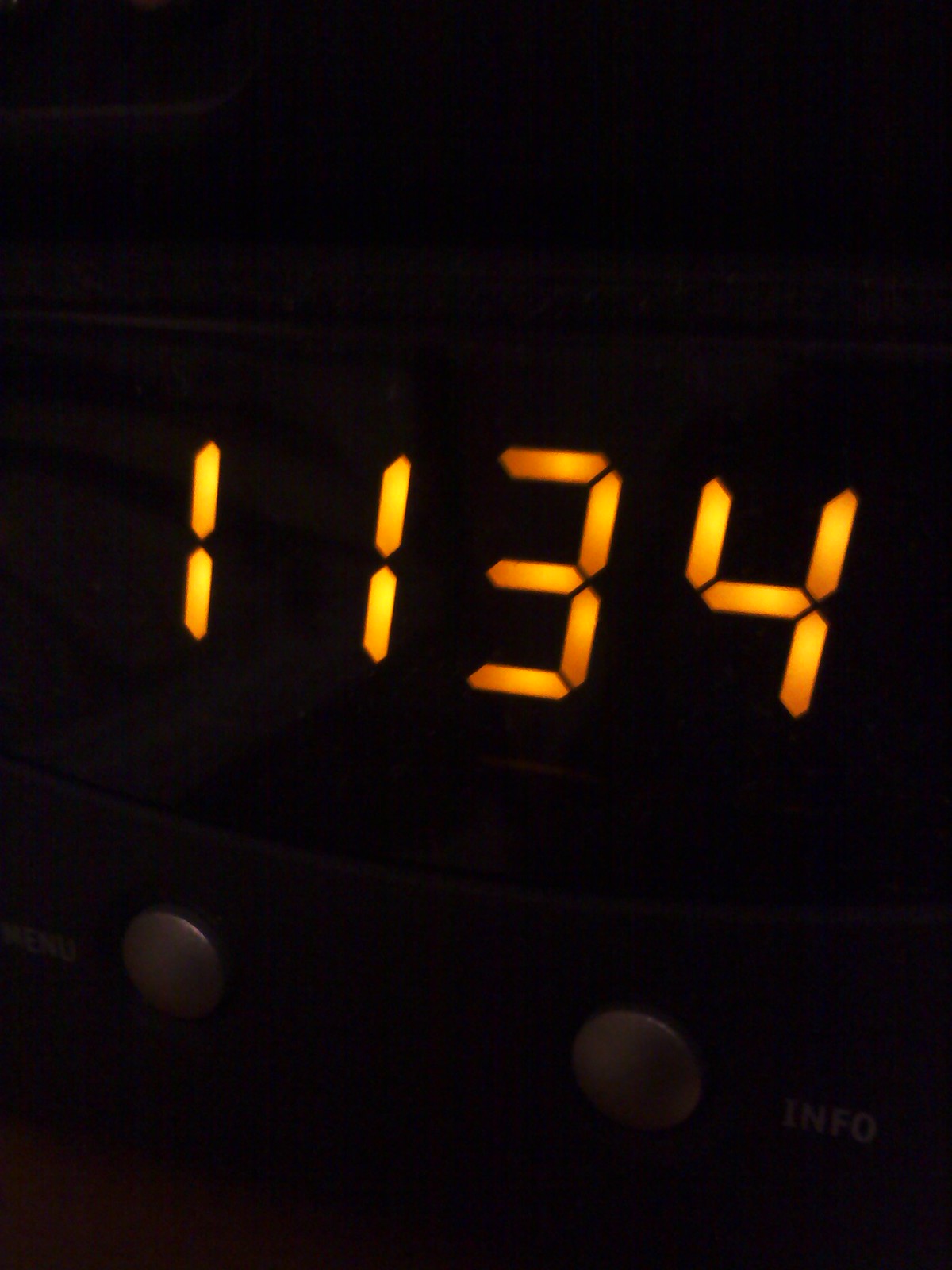Captured in a dark room or during nighttime, this image prominently features the face of a digital clock. The lack of background illumination emphasizes the clock's display, which glows in a vivid yellowish-orange hue, creating a stark contrast against the surrounding darkness. The time displayed is "1134," though the traditional center colon that typically separates hours and minutes is notably absent. Below the bright numbers, two faint silver dials are visible, likely integral components of the clock’s interface. Adjacent to these dials, the words "menu" and "info" are subtly discernible, hinting at additional functionalities of the device. The image is predominantly focused on the time display, making the "1134" stand out prominently at the center.